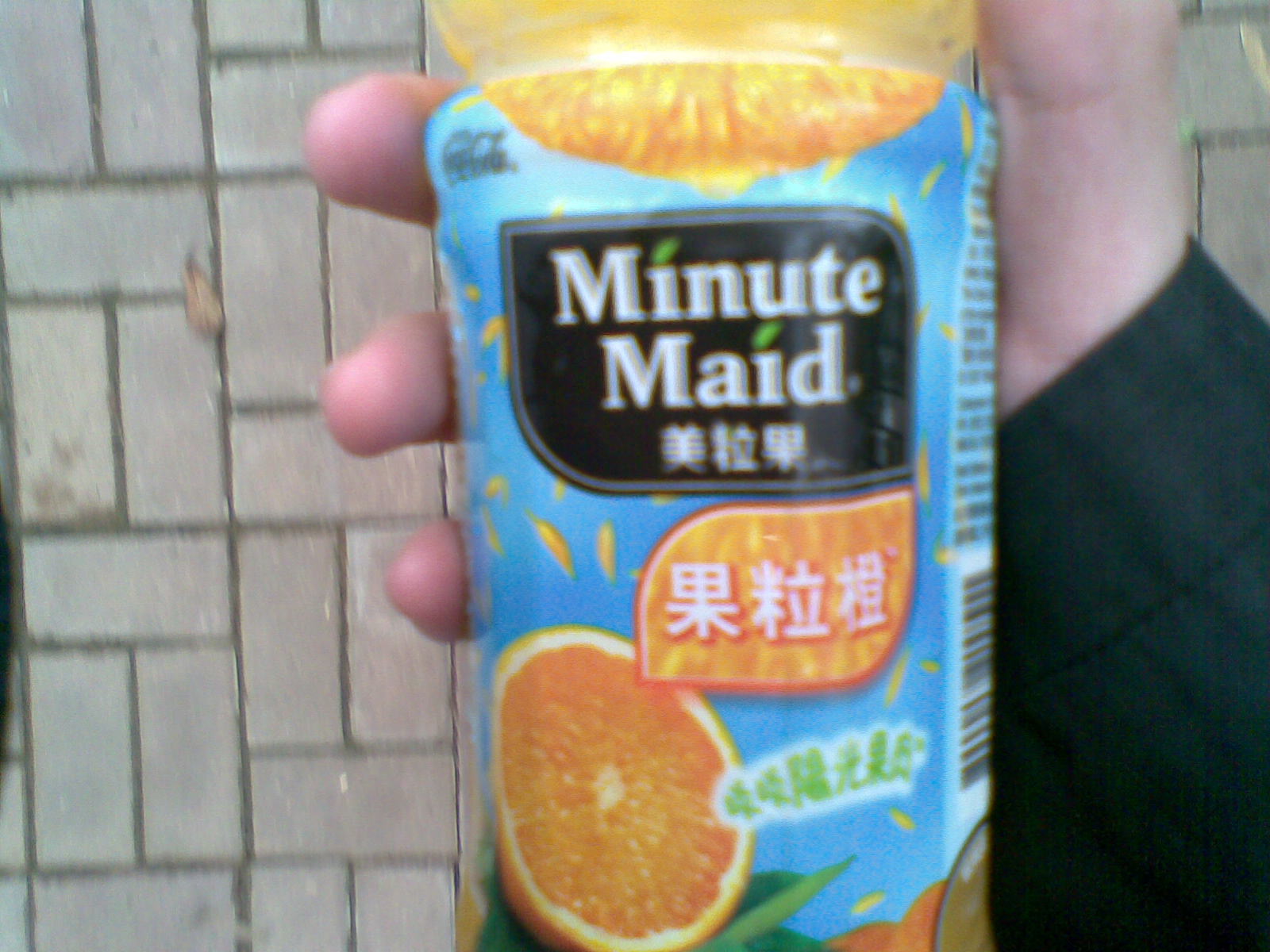The photograph, taken outdoors, features the right hand of a person of European descent, clad in a black long-sleeved shirt, holding a plastic bottle of Minute Maid orange juice. The bottle is prominently colored blue with a distinct black section displaying "Minute Maid" in white text. Below this, there are three Asian characters, likely Chinese, with an orange section highlighting an image of a half-sliced orange. The bottom part of the label includes additional Chinese characters and a number starting with "44." The angle of the shot is from above, capturing the thumb and tips of three fingers gripping the bottle, with the backdrop consisting of a gray, brick masonry ground and a hint of a stone wall in the background.